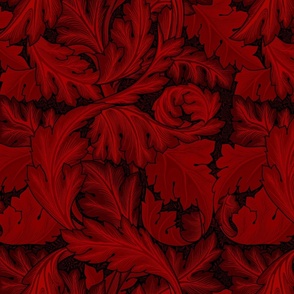The image depicts a detailed and intricate pattern, featuring a rich display of intertwined red leaves against a subtle black background. The pattern is reminiscent of a textured canvas or possibly wallpaper, with the black background lending a velvet-like appearance, enhancing the contrast with the dark burgundy leaves. These leaves, varying slightly in shade to provide depth and interest, dominate the image, curling and branching out in a harmonious and flowing design. Among the clustered leaves, there are occasional rounded objects with jagged edges and vertical cracks adding a layer of complexity to the composition. The overall effect is a strikingly rich visual marked by the interplay of the dark red hues against the sparsely visible black background, creating a captivating and somewhat mysterious pattern.